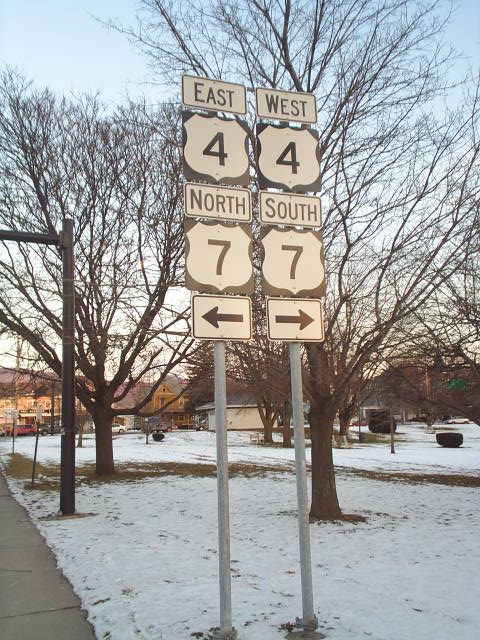This vertical, rectangular photograph depicts an outdoor scene during late afternoon on a winter day. The entire ground is primarily covered with a thin layer of snow, with a bit of dirt peeking through. The sky is a clear blue with some white patches. Dominating the center of the image are two tall, grayish-silver poles, each adorned with multiple traffic signs. The left pole features four white rectangular signs with black borders: from top to bottom, the signs read "EAST," display the number 4 in a curly-cued square, read "NORTH," display the number 7, and point left with an arrow. The right pole mirrors this pattern with signs that read "WEST," also displaying the number 4, read "SOUTH," display the number 7, and point right with an arrow. Surrounding the poles, snow-covered ground extends to several large, leafless trees, their brown trunks and branches stretched out in various directions. In the back of the scene, numerous buildings of varying colors—white, brown, and light brown—are visible, along with a few scattered cars to the left side. Additional street signs and poles pepper the background, contributing to the urban landscape.